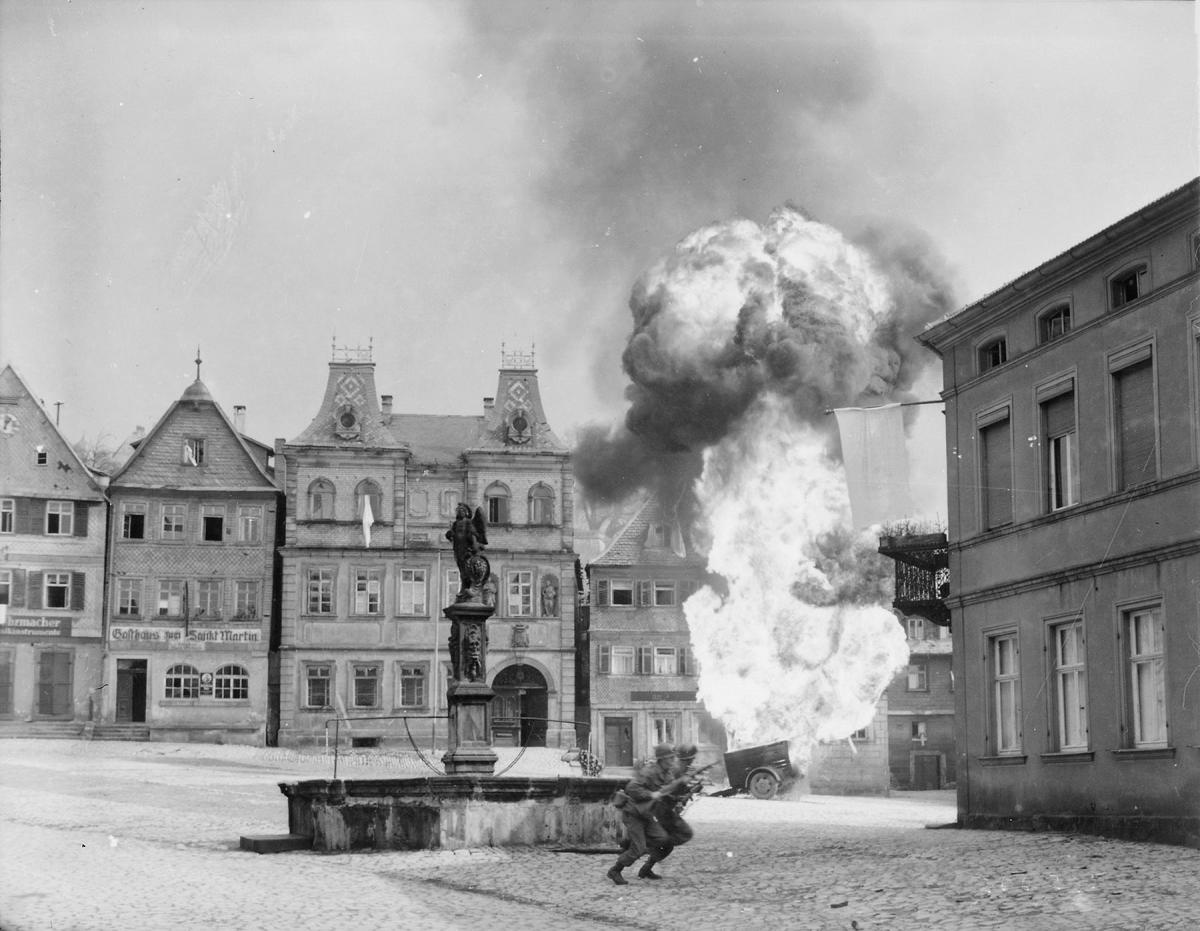An evocative black and white photograph captured during a wartime scene in the heart of a town. At the center stands a prominent statue atop a round base, likely a fountain, which serves as the focal point of the town square. Surrounding the square are buildings with a stone facade, displaying storefronts on the ground level and residential spaces above. In the lower center of the image, two soldiers are seen running side by side towards the right, each gripping their weapons firmly. To the right side of the central square, an explosion erupts from the ground, sending up a pillar of smoke in a mushroom-like shape, adding a dramatic and somber tone to the historical context of the photograph.